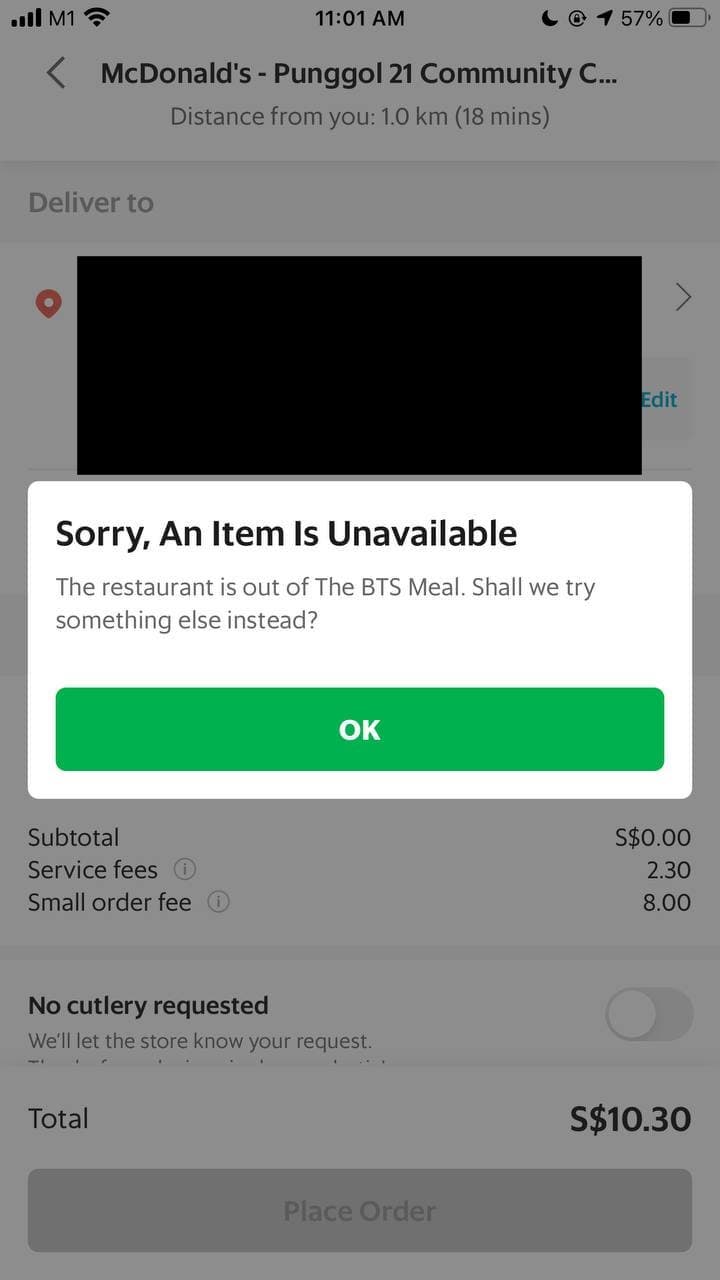**Caption:**

In this vertically-oriented smartphone screenshot, the background appears beautifully faded, drawing attention to a central horizontal rectangle. At the upper left corner of the image, the usual smartphone status indicators are displayed: signal strength, 'M1,' Wi-Fi signal, and the time, 11:01 a.m. Positioned centrally at the top, icons for the moon, a lock, and a battery indicator showing 57% charge are visible.

The prominent section in the middle features text in black: "McDonald's - Punggol 21 Community Club." Beneath, it notes, "Distance from you: 1.0 kilometers (18 minutes)." The instruction to "Deliver to" is followed by what should be a map, but it is instead represented by a black box. 

Lower in the screenshot are details of the order: 
- Subtotal: $0.00
- Service fees: $2.30
- Small order fee: $8.00
- No cutlery requested

The note confirms that the store has been informed about the lack of cutlery request, which is toggled off, leading to a total cost of $10.30. A button to "Place order" is present but grayed out, indicating it's inactive.

Prominently in the center of the image, a white rounded rectangle conveys in bold black text: “Sorry, an item is unavailable.” Below, in less bold text, it clarifies: “The restaurant is out of the BTS meal. Shall we try something else instead?” Directly underneath this message, a green button contains the text “OK” in white, meant to be pressed as the next action step.

**Image Description:** In this smartphone screenshot, we're given a snapshot of an incomplete food delivery order from McDonald's, with clear indicators of unavailable items and the option to select alternatives. Despite the faded background, every essential detail about the order, fees, and smartphone status is rendered in clear, easily readable segments, punctuated by the alert about the unavailable BTS meal.